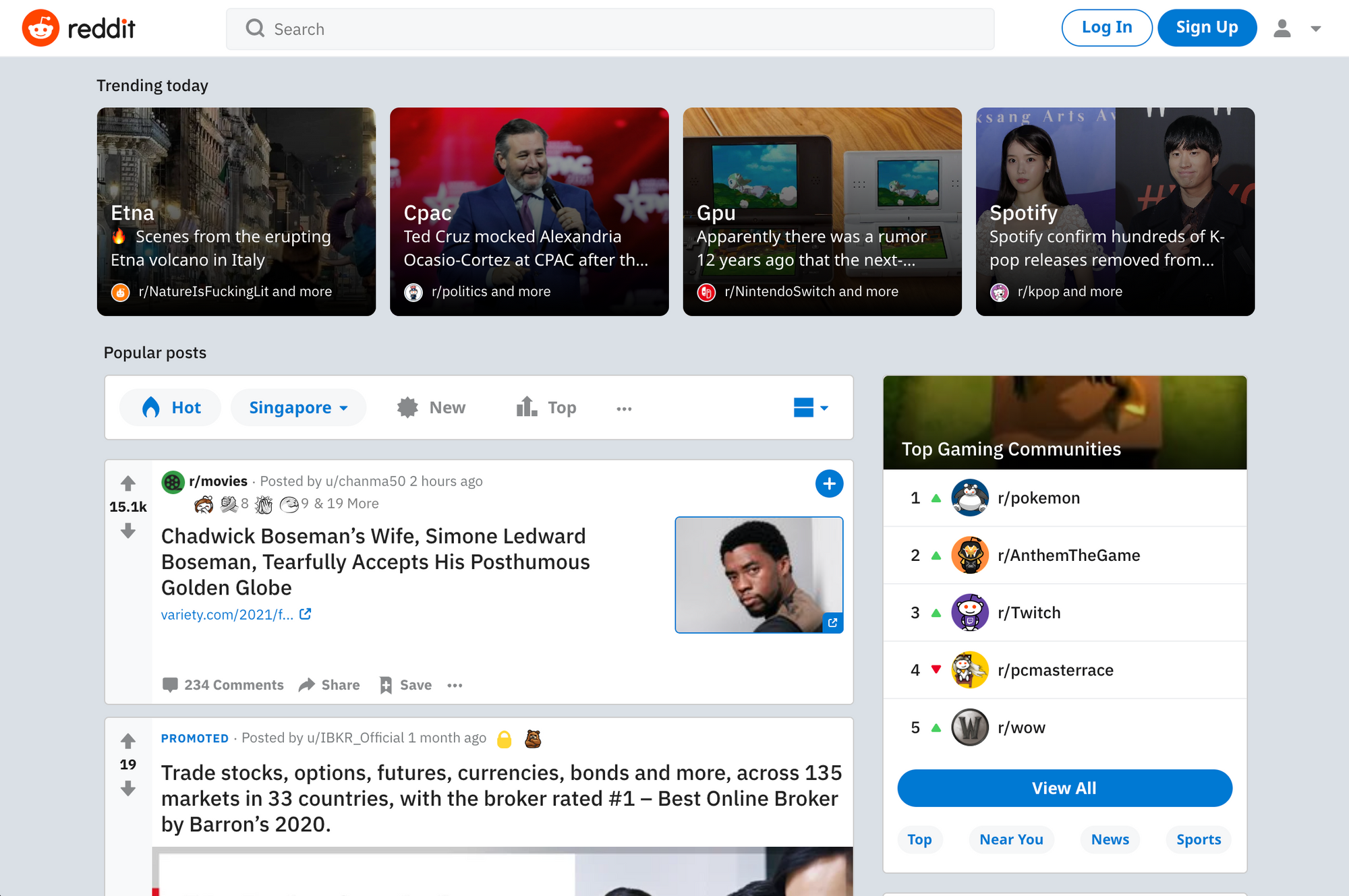The image showcases a Reddit news aggregator page. The distinctive Reddit branding is noticeable in the upper-left corner, featuring the Reddit logo—an orange circle with a white alien face inside. Adjacent to the logo, the word "Reddit" is displayed in black font. Extending to about two-thirds of the page's width, a gray rectangular search bar is present, containing a small magnifying glass icon and the word "search" in gray font. To the right of the search bar are two oval buttons: a white one with blue outline and blue text reading "Log In," and a blue one with white text reading "Sign Up." Additionally, there's a small social media icon accompanied by a down arrow.

Beneath this header section, the page dives into an aggregation of various news items. At the top, there's a "Trending Today" section featuring four small image icons, each representing a separate trending news story. Below this, the typical Reddit navigation menu is displayed, including options such as "Hot," "New," and other sorting buttons commonly found across Reddit posts for easy navigation and categorization of news content.